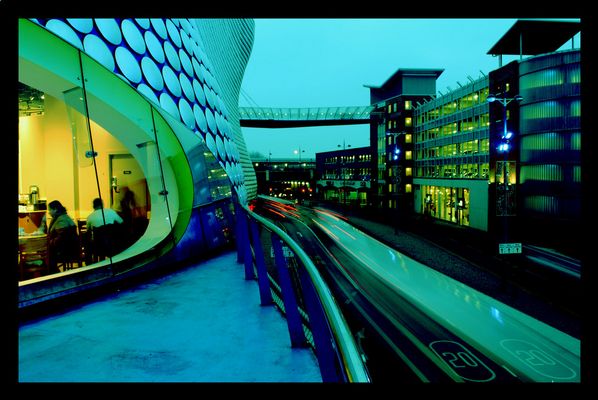The image depicts a futuristic cityscape with a prominent, uniquely shaped building on the left side of the frame. This building features an oval-shaped window in the middle-left portion, with people visible inside, likely in a restaurant or office setting. Its exterior is adorned with circular tiles that are white with a slight bluish hue, and darker blue outlines around each tile. The building's surface also displays horizontal stripes, which appear vertical due to the structure's curvature, giving it a scaled, almost sci-fi appearance.

To the right of the picture, a pair of tracks marked with the number 20 can be seen, one black and the other white. There is an impression of motion on these tracks, suggesting a moving vehicle or train. Spanning over the tracks is an enclosed walkway connecting two long, tall buildings that stretch into the background, hinting at urban density. The sky and upper part of the picture have a distinct bluish tinge, resembling the look of an image on a TV screen, while the ground area between the buildings appears to be concrete. Despite the nighttime setting, the scene is vibrant, showcasing a blend of illuminated modern architecture and bustling city life.